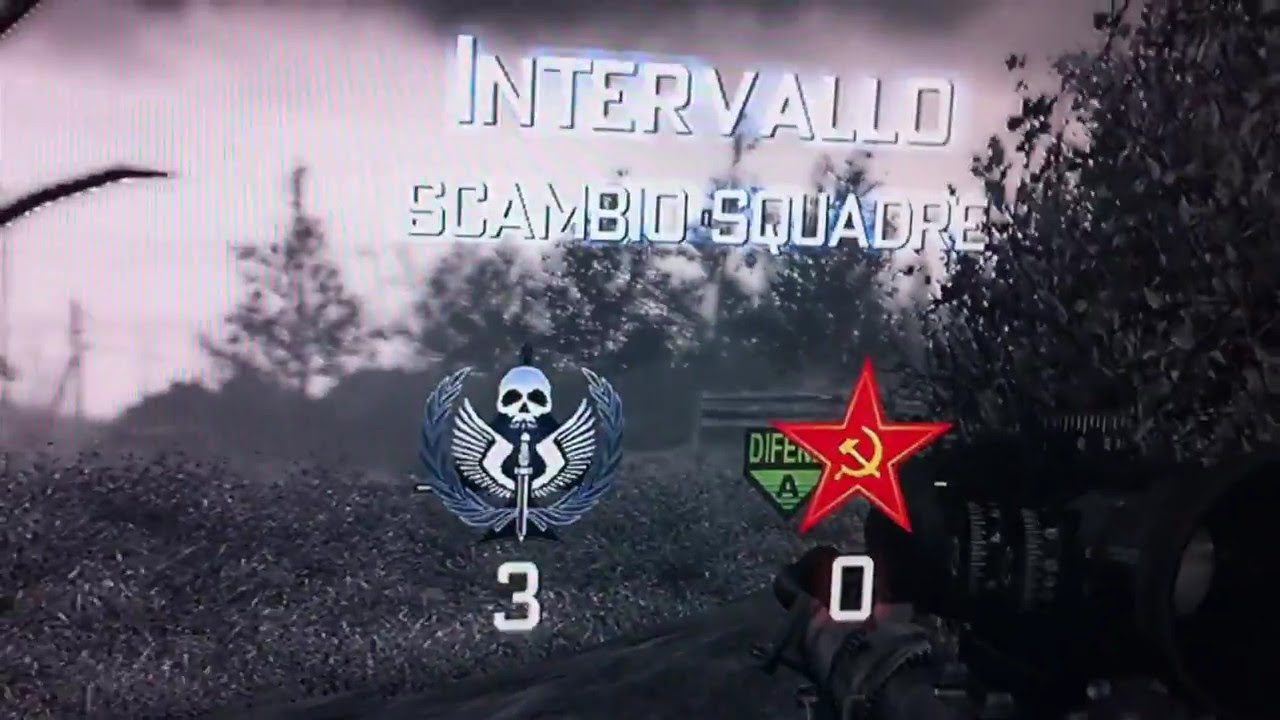The image appears to be a screenshot from a video game, showing a dark, shadowy landscape with dead trees, dirt roads, and bushes in black and white. Dominating the center are the words "Intervallo Scambio Squadre" in digital lettering. To the left, there's a black and white emblem featuring a skull with wings and a sword, bearing the number three below it. On the right, there's a red star with a gold hammer and sickle, which has a zero underneath it. Only the red star stands out in color against the otherwise monochromatic background. A sniper rifle is visible in the bottom right corner. This screenshot seems to depict a scene where one team, symbolized by the skull emblem, is leading with a score of three, while the opposing team, represented by the red star, has a score of zero.